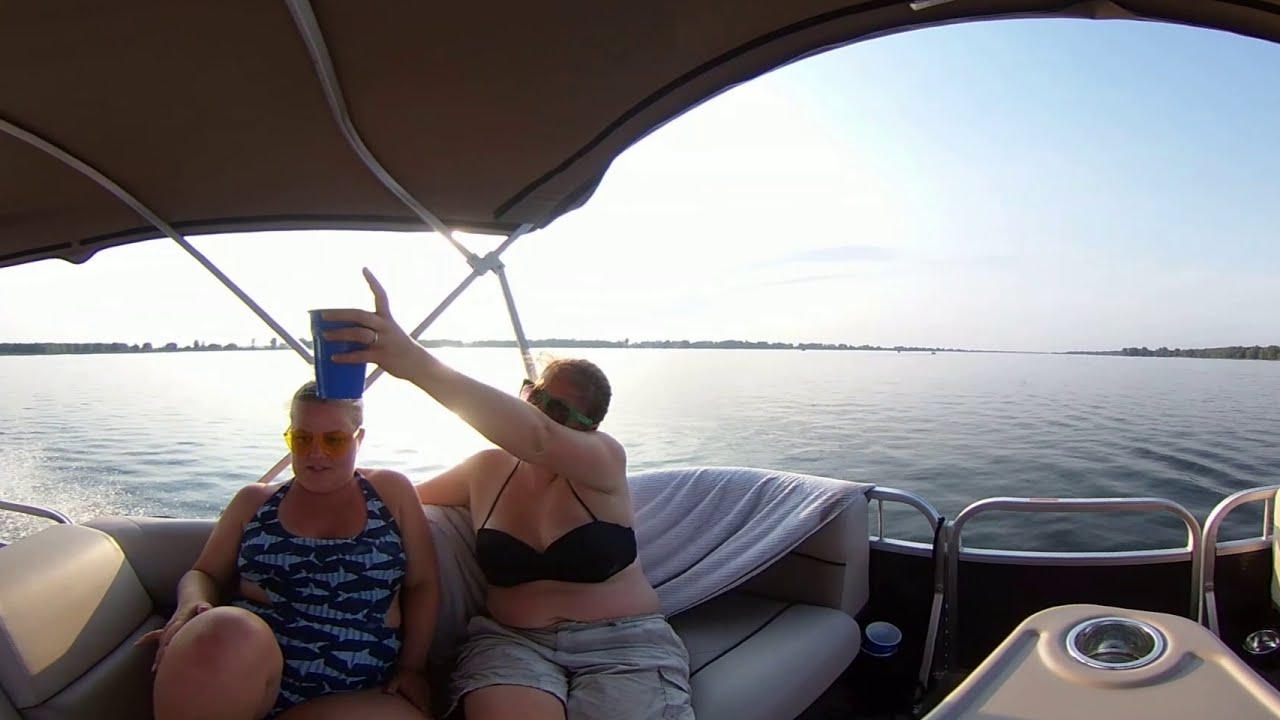In the image, two women are seated at the back of a pontoon boat on a calm lake under a cloudless, sunny sky. The boat features a stretched, brown roof screen providing a casual, relaxed vibe. Both women, seated on a soft, white leather chair, are wearing sunglasses—one with yellow aviators and the other with green-framed black shades. The woman on the left, who has short hair and is grinning while touching her knee, is dressed in a blue one-piece bathing suit adorned with shark patterns. The woman on the right, also short-haired, is wearing a black bikini top paired with khaki cargo shorts and holds a blue solo cup aloft, as if toasting. The serene water reflects sunlight, and distant tree-lined or building-dotted horizons complete the tranquil lake scene.